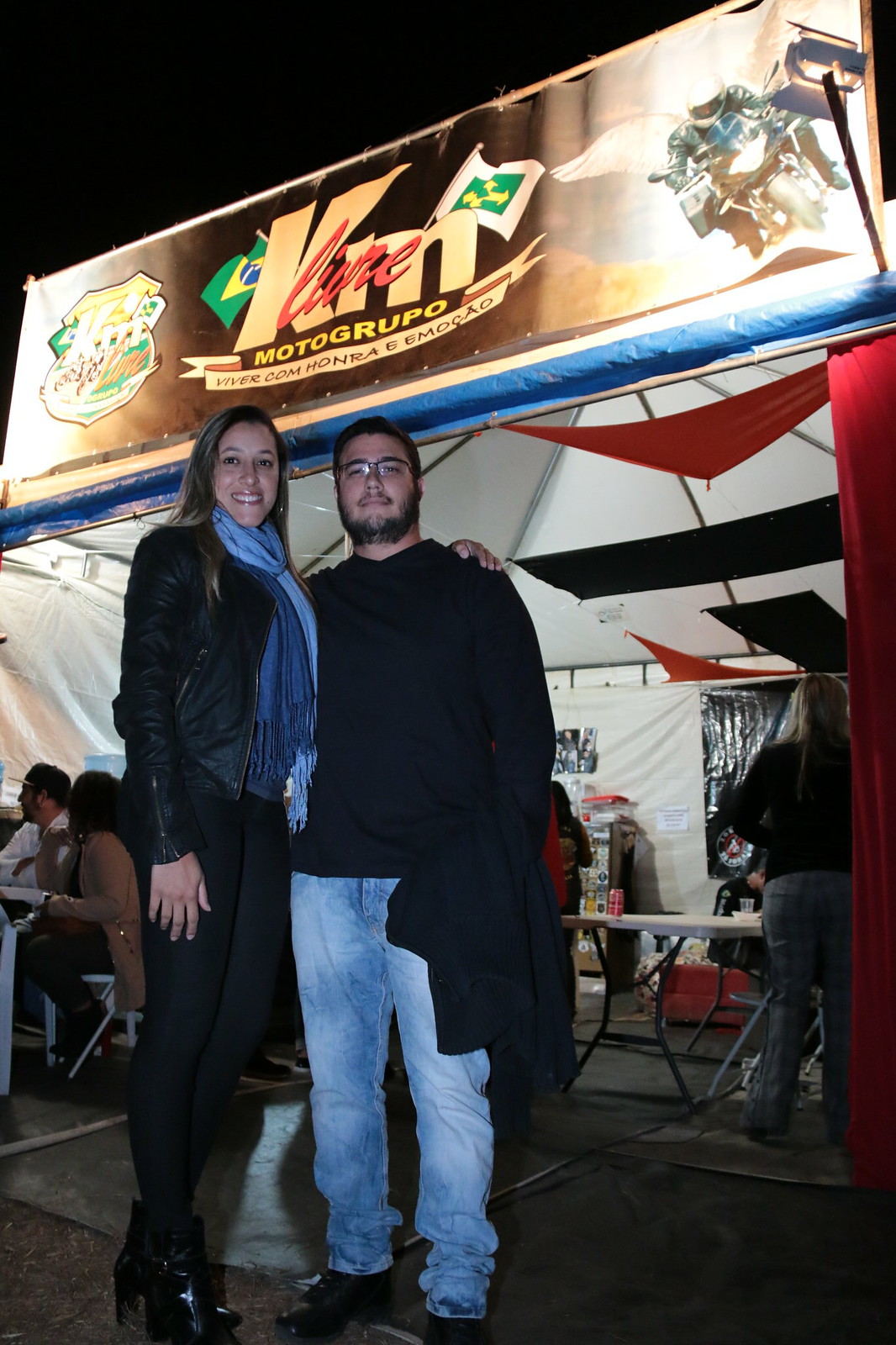In this photograph, a young couple is standing in front of a food stall with a sign that reads "Moto Grupo" above them, possibly indicating a connection to motorsports. The woman on the left, a white woman in her 20s, is dressed stylishly in a black leather jacket, tight black pants, black boots, and a decorative blue scarf around her neck. She smiles warmly at the camera. The man on the right, also white-skinned, sports black hair, glasses, and a thick neck beard that almost forms a mustache. He wears a black long-sleeve shirt, light blue jeans, and black shoes. He holds a black jacket in his left hand. The couple stands in front of a pop-up tent, with people seated behind them around a white folding table. The tent is adorned with Brazilian flags and imagery of a sports bike on the right side of the image.